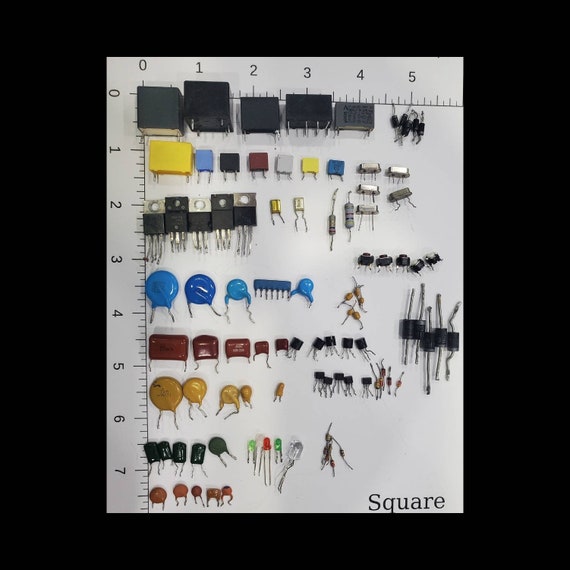This image depicts a white piece of paper bordered with a ruler scale on the top and left sides. The horizontal ruler spans from 0 to 5 inches and the vertical one from 0 to 7 inches. The page contains various electronic components such as electrodes, nodes, and capacitors, each with distinguishable colors and metallic wires protruding from them. These components, which include colors like dark gray, yellow, blue, black, maroon, white, and mustard, are arranged in rows. Notably, some components are encased in shiny plastic coverings, resembling Christmas lights, and others are small black boxes with silver wires. At the bottom right corner of the paper, the word "square" is clearly printed in black serif text. The entire setup is positioned against a black backdrop.